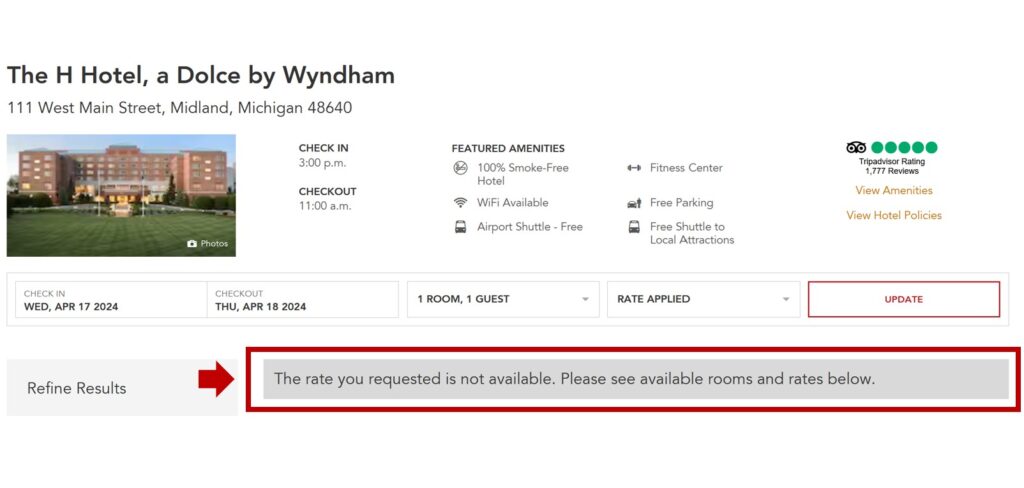### Caption:
In this screenshot from a website, set against a solid white background, the upper left corner features dark bold text reading "The H Hotel, a Dolce by Wyndham". Directly below it, in smaller gray text, is the address "111 West Main Street, Midland, Michigan 48640". Below the address is a colored photograph of the hotel façade, which appears to be approximately five stories high, with a sprawling green lawn in the foreground.

Beneath the photo, there are several informational boxes: 
- **Check-in:** Wednesday, April 17th, 2024
- **Check-out:** Thursday, April 18th, 2024

To the right of these boxes, bold text displays "One room, one guest" with a down arrow for a dropdown menu. Next to this, another dropdown box labeled "Rate applied" is also present. Finally, on the far right, there's a prominent red button labeled "Update".